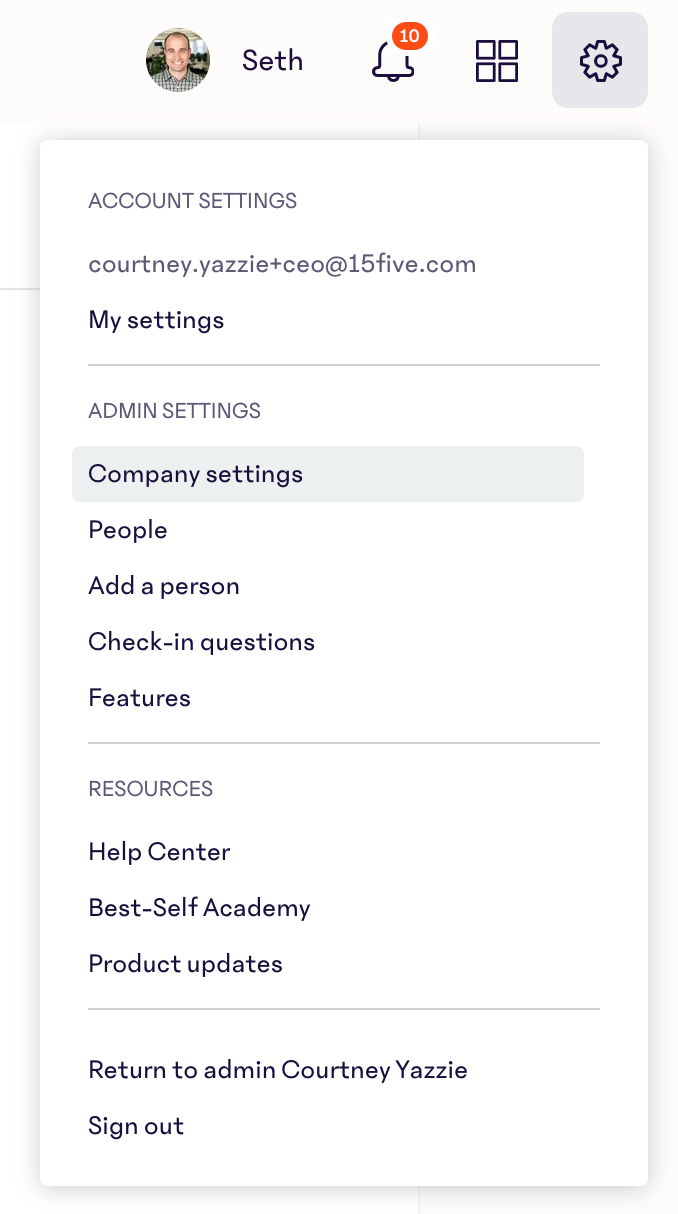The image presented unveils a structured user interface with a predominantly white background. Positioned at the top is the profile picture of a white Caucasian individual, identified as "Seth" by the adjacent black-font name tag. Next to Seth's name, there's an image of a bell inside an orange circle, marked with the number 10 in white, likely indicating notifications.

Below the profile image and notifications icon, there are four conjoined grey squares forming a single unit, followed by another grey-outlined square containing the settings logo. Beneath this, a section on a white background features a grey-font label "Account Settings". Just under this heading, the email address "Courtney.yazzyplusceoat155.com" is displayed, followed by a "My Settings" option with a grey dividing line underneath, and then an "Admin Settings" option.

In a grey box with black font, "Company Settings" is listed, and the structure continues with the following items sequentially: "People," "Next Person," "Add a Person," "Check-in Questions," and "Features." A grey line separates this segment from the next.

Below the line, the section "Resources" is listed, encompassing "Help Center," "Best Self Academy," and "Product Updates," arranged in descending order. Another grey line segments the end portion which includes options to "Return to Admin Courtney Yazzy" and "Sign Out" at the bottom.